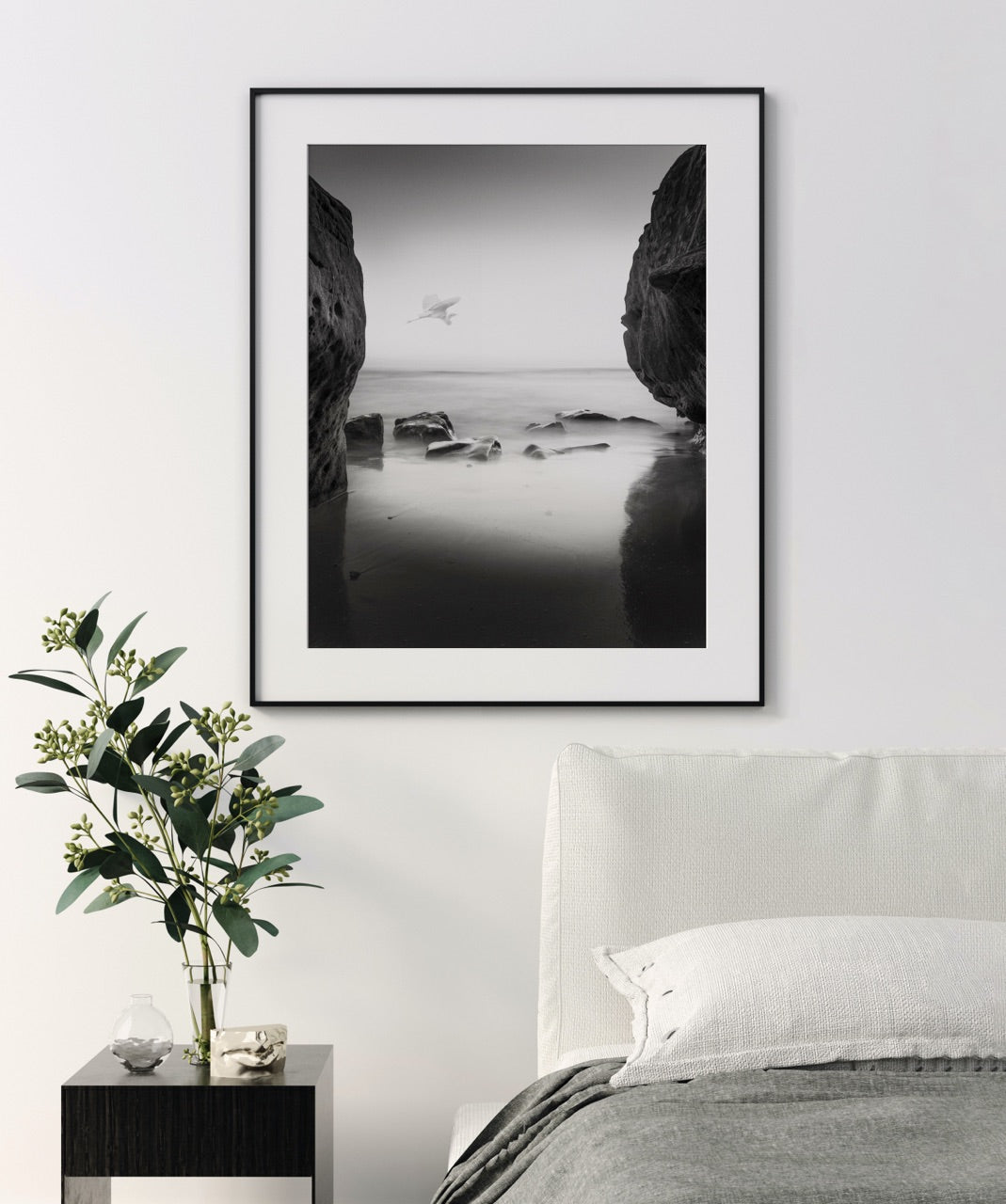The image depicts a serene bedroom with a light gray wall, featuring a bed in the lower right-hand corner. The bed has a white linen headboard, adorned with a gray blanket and a white pillow. Adjacent to the bed is a small, dark brown wood nightstand. On the nightstand, there is a light beige glass decorative object, a small clear glass bud vase, and a medium tall clear glass vase containing stems with large dark green leaves and light green buds.

Hanging above the bed is a striking black-and-white photograph framed with a thin dark frame and a wide border. The photograph captures a beach scene with two large rocks flanking the sides, where the ocean meets the wet sand. A bird is visible in the sky, enhancing the tranquil atmosphere of the scene. The image evokes a sense of calm and invites a closer look at the interplay between the natural elements depicted.